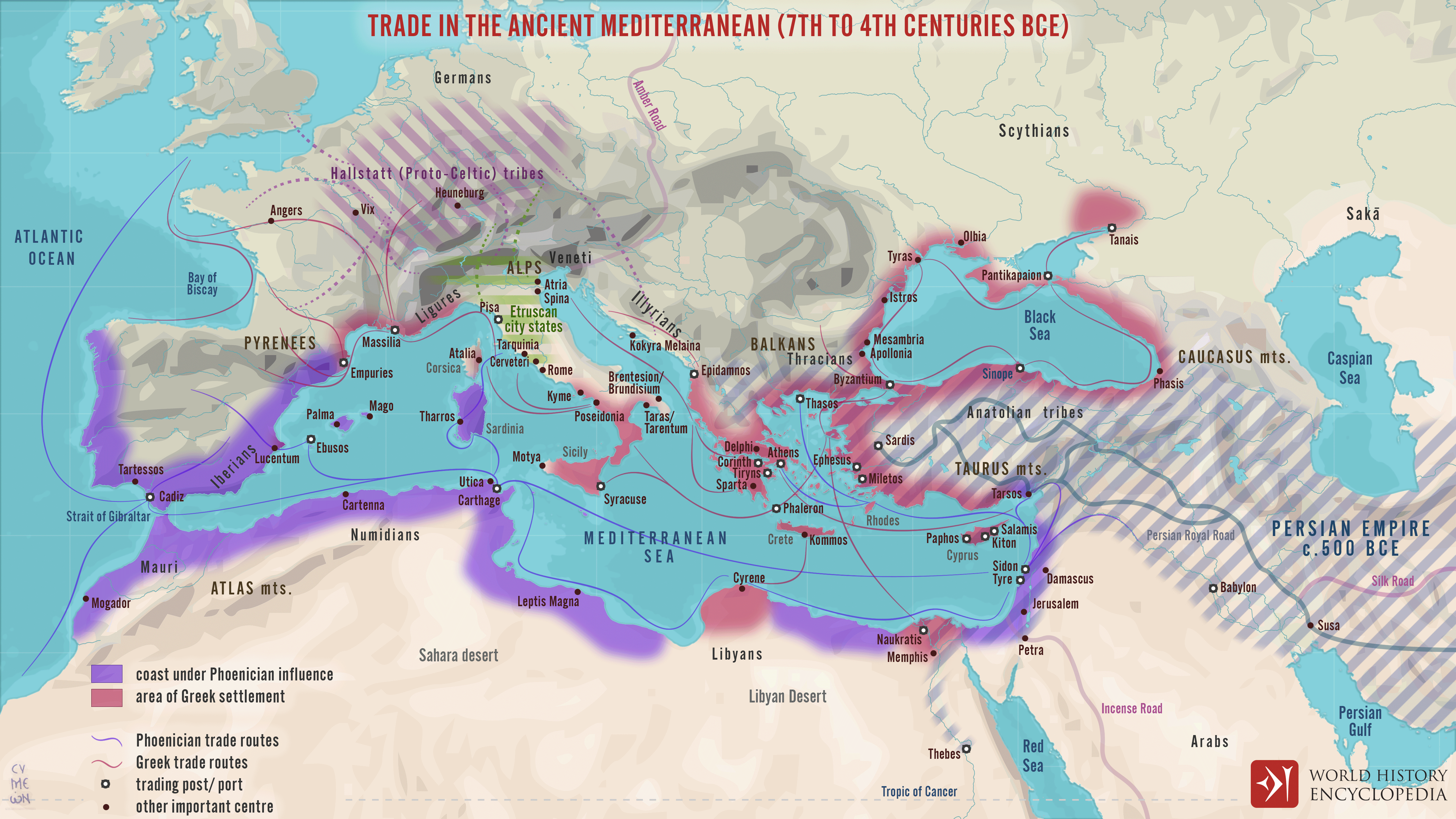The image is a detailed map titled "Trade in the Ancient Mediterranean (7th to 4th centuries BCE)" depicted in red text at the top. The map highlights the Mediterranean area and includes features such as the Mediterranean Sea in the center, the Atlantic Ocean in the top left corner, the Black Sea to the east, and the Caspian Sea. To the south, the map shows the Persian Gulf. The map also includes the northern parts of Africa and several ancient regions labeled, such as the Pyrenees, Germans, Scythians, Caucasus, and the Persian Empire.

The map uses color to indicate various trade routes and regions of influence. Purple shading highlights coastlines under Phoenician influence, with corresponding purple trade routes stretching across the map. Areas of Greek settlement and their trade routes are marked in pinkish red. A key in the bottom left corner clarifies these colors and their meanings. Additionally, in the bottom right corner, the map credits the "World's History Encyclopedia". This comprehensive depiction provides insight into ancient trade networks and settlements in the Mediterranean region.